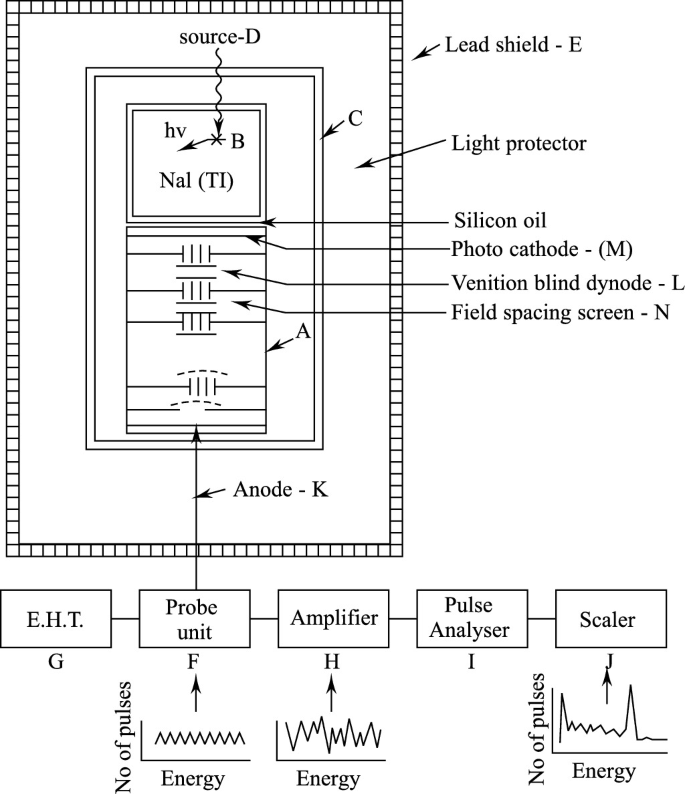The image is a detailed electrical schematic of an electronic device, featuring multiple interconnected components arrayed primarily within a large vertical rectangle. The schematic, rendered entirely in black text and simple shapes on a white background, includes numerous lines, squares, and rectangles with arrows pointing to specific parts. At the top are labeled components: "source-D," "lead shield-E," "HVB NALTIC," "light protector," "silicon oil," "photocathode-M," "Venetian blind dynode-L," "field spacing screen-N," "A," "anode-K," "EHT," "G," "probe unit," "F," "amplifier," "F," "pulse analyzer," "I," "scaler," "J," with repeated mentions of "number of pulses" and "energy."

Inside the main large rectangle, the components are laid out vertically from top to bottom: "lead shield," "light protector," "silicon oil," "photocathode," "Venetian blind dynode," and "field spacing screen." Below these are five smaller rectangles labeled "G," "F," "H," "I," "J," corresponding to "EHT," "probe unit," "amplifier," "pulse analyzer," and "scaler." These are connected to indicators for "energy" and "number of pulses," each depicted with zigzag waveforms akin to heart monitor graphs, emphasizing the pulse analysis function of the device. This intricate diagram highlights the connections and operational flow within the schematic, providing a clear overview of the device's structure and function.